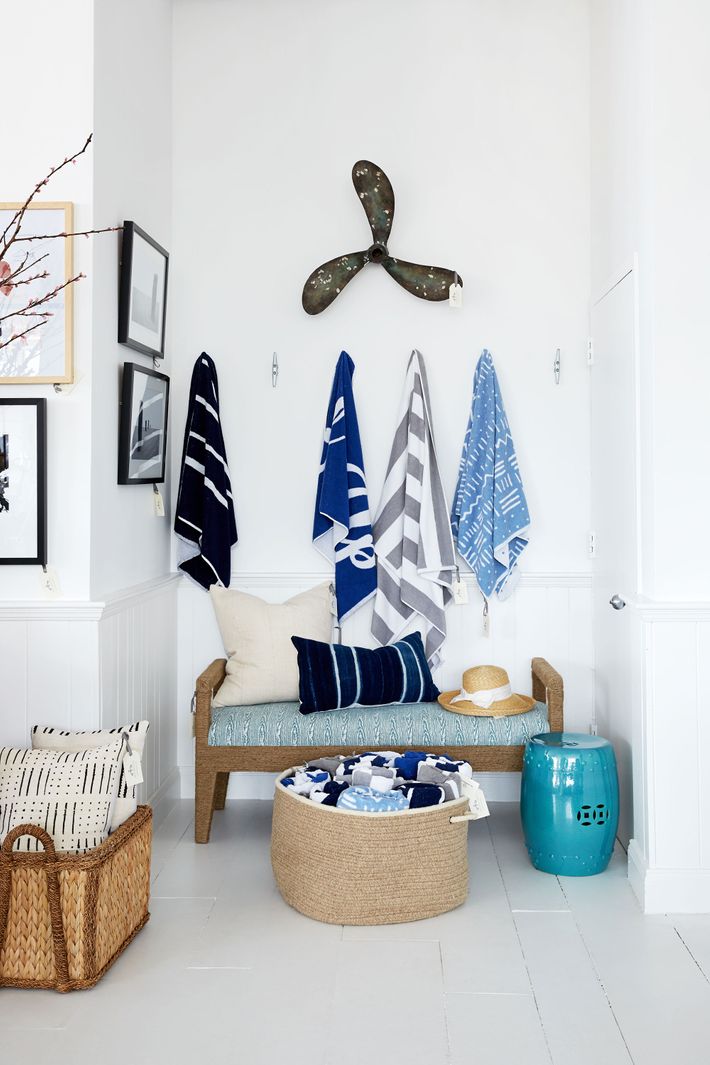The image depicts a cozy nook within a home, characterized by a recessed white wall serving as a charming backdrop. On this wall, there's a set of black and wooden-framed pictures, partially visible, adding a touch of personal flair. The focal point is a small wooden bench nestled within the cubby area, topped with a teal cushion, a pair of pillows—one white and one blue—and a sun hat. Surrounding the bench are six hooks, four of which are adorned with striped towels in various shades of blue, black, and gray. Above these, there's an eye-catching, three-blade propeller mounted on the wall. The floor features white wooden vertical panels, enhancing the room's airy aesthetic. Below the pictures, there's a wicker basket containing what appears to be white pillows or blankets. Another wicker basket and a blue bin are positioned on the floor to the right, presumably for additional storage. A mix of color tones—blue, black, white, and a hint of brown from the baskets—harmonize the space, creating a welcoming, nautical-inspired entryway.